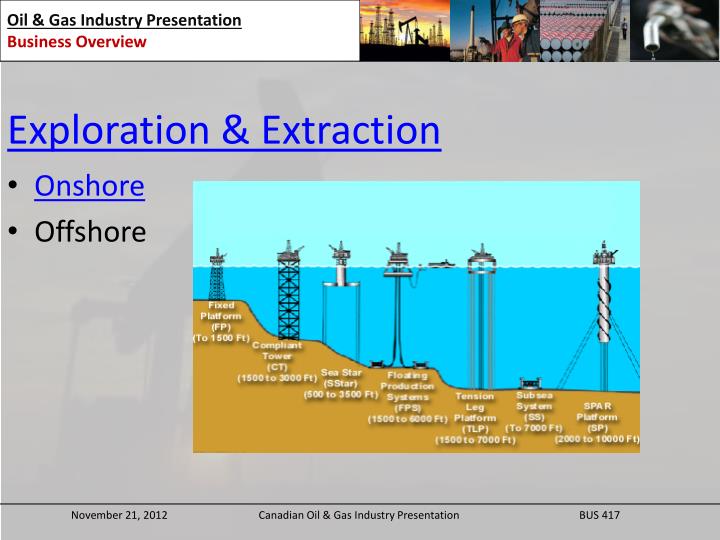The slide is part of an oil and gas industry presentation and includes multiple elements. In the top left corner, "Oil and Gas Industry Presentation" is prominently underlined in black text on a white background, followed by "Business Overview" in striking red text underneath. Adjacent to this, on the right side, are four photographs: one of an oil digger, one of two engineers in hard hats, an image of stacked cylinders likely in a factory setting, and another depicting a tap with liquid dripping out. Below the photos, a large gray section contains blue underlined text reading "Exploration and Extraction," followed by bullet points in blue and black for "Onshore" and "Offshore," respectively. To the right, a detailed schematic illustrates various types of oil rigs in different positions on the seafloor, including Fixed Platform (FP) up to 1500 feet, Compliant Tower (CT) from 1500 to 3000 feet, Sea Star (S Star) from 500 to 3500 feet, Floating Production System (FPS) from 1500 to 6000 feet, Tension Leg Platform (TLP) from 1500 to 7000 feet, Subsea System (SS) up to 7000 feet, and Spar Platform (SP) from 2000 to 10,000 feet. The bottom left corner of the slide notes the date "November 21st, 2012," identifying it as a "Canadian Oil and Gas Industry Presentation," and the course or project identifier "BUS 417" is located in the bottom right.